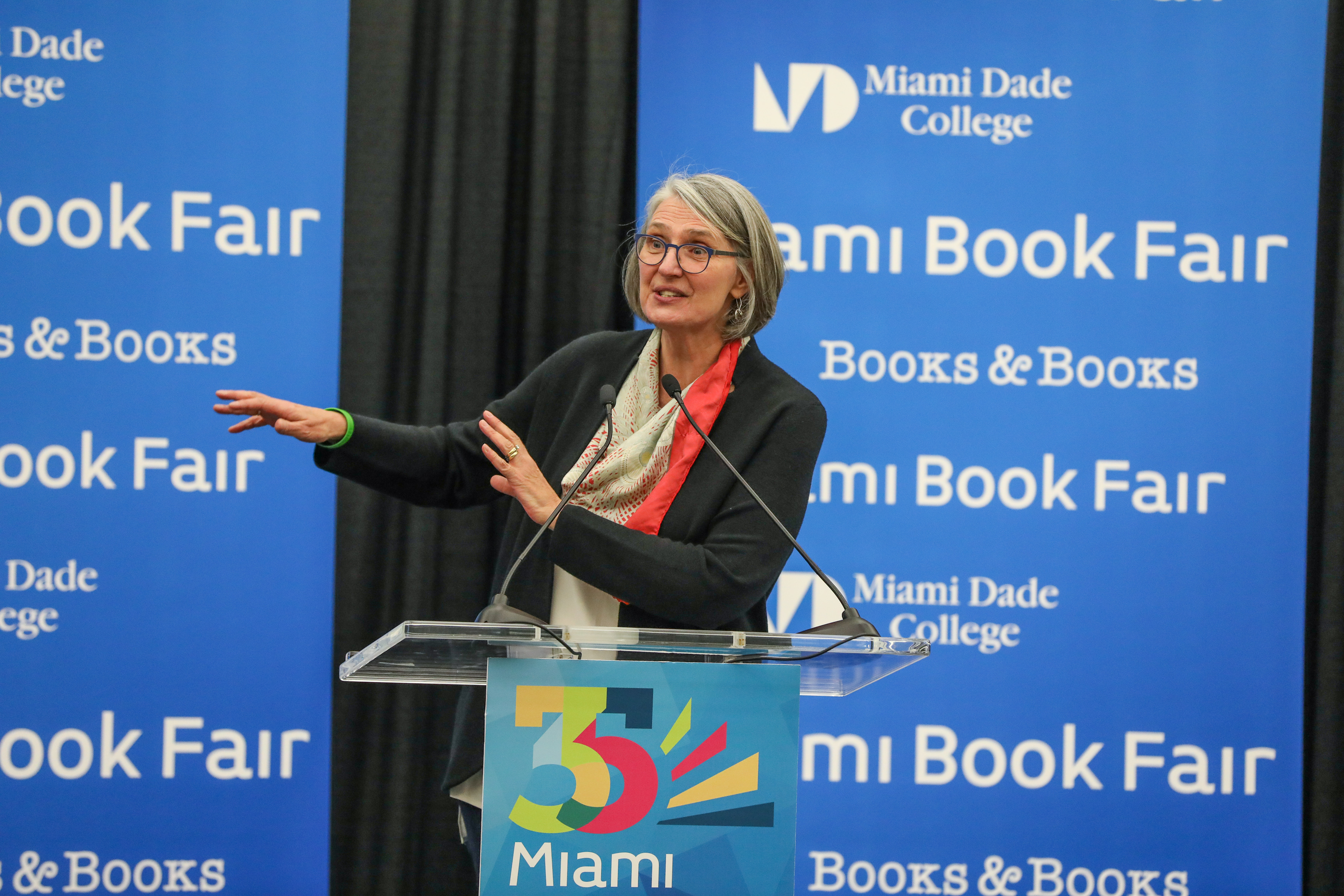The image is a horizontally aligned rectangular picture of a woman standing at a glass podium. The podium prominently features a multicolored "35" logo at the front, with the number blending from yellow, light green, dark blue, peach red, light blue, to dark green, and trailing lines of similar colors extending outward. Below the "35," it reads "Miami" in white against a light blue background. The podium is equipped with two protruding black microphones.

The woman, appearing to be in her 40s or 50s, has short bobbed gray hair with hints of brown, and is wearing black-framed glasses. She is dressed in a black cardigan over a tan blouse, accented with a red and cream-colored scarf. She is animatedly speaking, with both hands gesturing expressively in front of her. A wedding ring is noticeable on her hand.

Behind her on the stage is a black curtain, flanked by two large vertical blue banners on either side. These banners bear repeating text in white, starting with "Miami Dade College" at the top, followed by "Miami Book Fair," "Books and Books," and then repeating "Miami Dade College," "Miami Book Fair," and "Books and Books" again. The woman's presence partially obscures the banners.